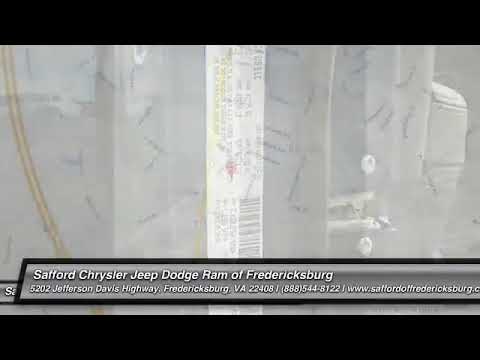The image appears to be the final frame of a car commercial set at Safford Chrysler Jeep Dodge Ram of Fredericksburg. Dominating the image is a partially faded and pixelated vertical VIN barcode, seemingly captured through a window. The QR code is visible, but the VIN number itself is indecipherable. Subtle streaks of gray extend across the image, adding to the faded effect. On the right side, you can faintly make out portions of the car's leather seats. At the bottom of the image, enclosed in a gray text box with a black border, white text displays detailed dealership information: "Safford Chrysler Jeep Dodge Ram of Fredericksburg, 5202 Jefferson Davis Highway, Fredericksburg, VA 22408" along with the phone number "1-888-544-1812" and a partially cut-off website "www.saffordfredericksburg.c...". The composition features medium-thick black borders at both the top and bottom edges.